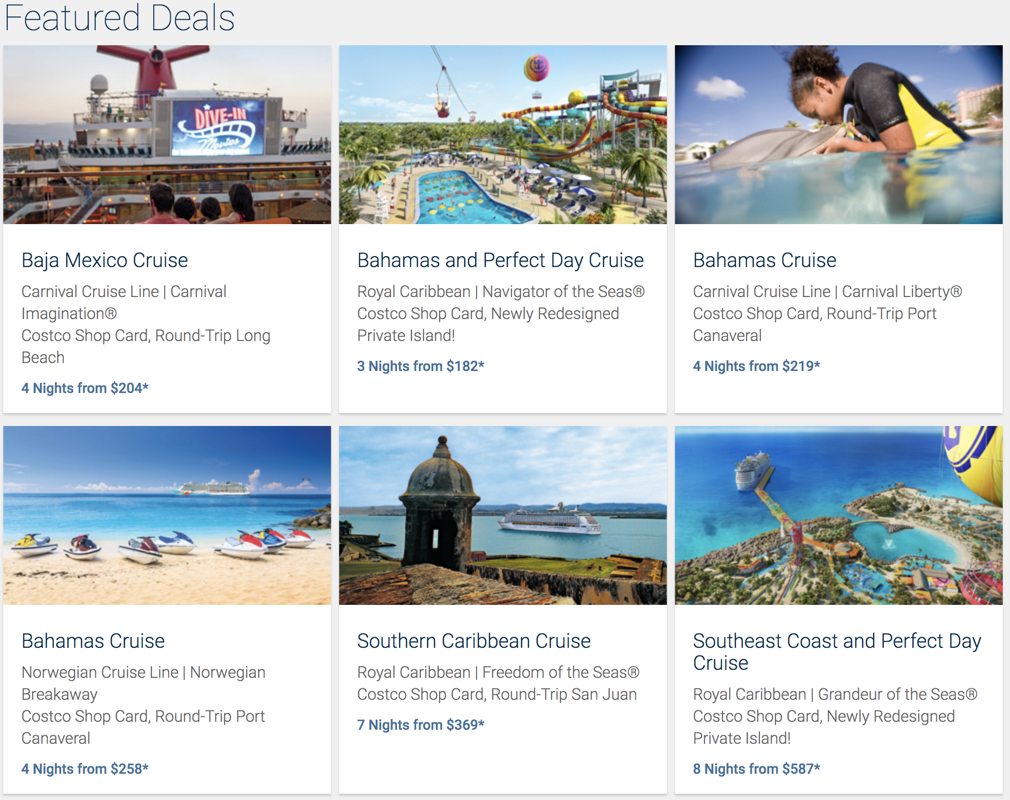This screenshot showcases an advertisement for Carnival Cruise Line deals. The upper left corner features a gray background with white and black text that reads "Feature Deals." The main content includes a series of cruise offers accompanied by images of a cruise ship with a prominent red funnel. Here are the details of the advertised deals:

1. **Baja California/Baja Mexico Cruise**
   - Duration: 4 nights
   - Price: $204

2. **Baja Perfect Day Cruise**
   - Duration: 3 nights
   - Price: $182

3. **Bahamas Cruise**
   - Duration: 4 nights
   - Price: $219

4. **Bahamas Cruise**
   - Duration: 4 nights
   - Price: $258

5. **Southern Caribbean Cruise**
   - Duration: 7 nights
   - Price: $369

6. **East Coast/Southeast Coast and Perfect Day Cruise**
   - Duration: 8 nights
   - Price: $587

The screenshot appears to be outdated given the unusually low prices for these cruises. The sender of the screenshot, Matt, expressed gratitude to his team for their efforts and speculated about the possibility of adding more deals due to the holiday season.